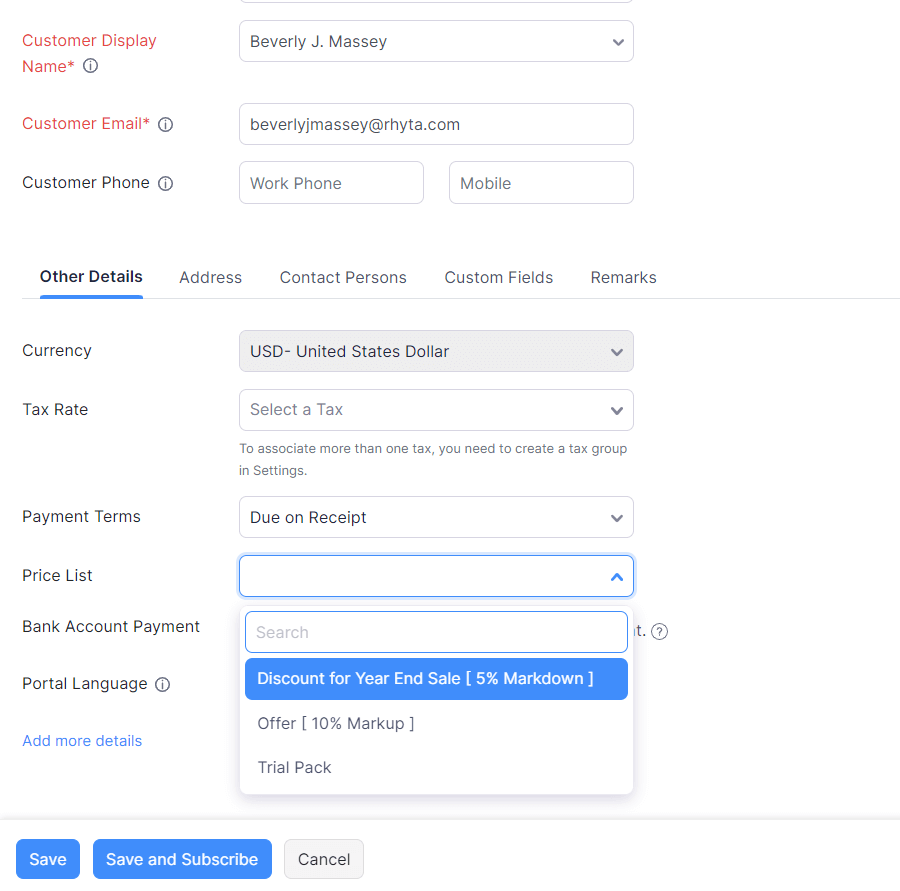This image depicts an online form with a variety of fields and options that require detailed user input. The form begins with the "Customer Display Name" field, highlighted in red, alongside an icon resembling an eye for visibility options. In this instance, the name "Beverly J. Macy" has been entered.

Next is the "Customer Email" field, also marked in red, displaying "Beverly J. Macy" again. The "Customer Phone Number" section allows for the input of either a work or mobile phone number.

The form includes several sections categorized under "Other Details," "Address," "Contact Persons," "Custom Fields," and "Remarks." Within these, the currency is set to U.S. dollars, and there is an option to select a tax rate from a dropdown menu. An informative note indicates that to associate more than one tax rate, a tax group must be created in the settings.

Payment terms are specified as due on receipt, with this option available via a dropdown menu. Users are prompted to enter a list price and have the ability to search for a bank account for payment.

Additionally, there is a section for discounts related to year-end sales, featuring a 5% markdown and a 10% markup offer. A trial pack option is also mentioned. Further details can be added, including selecting a portal language.

The form provides actionable buttons at the end: a blue "Save" button, a longer blue "Save and Subscribe" button, and a gray "Cancel" button for user convenience.